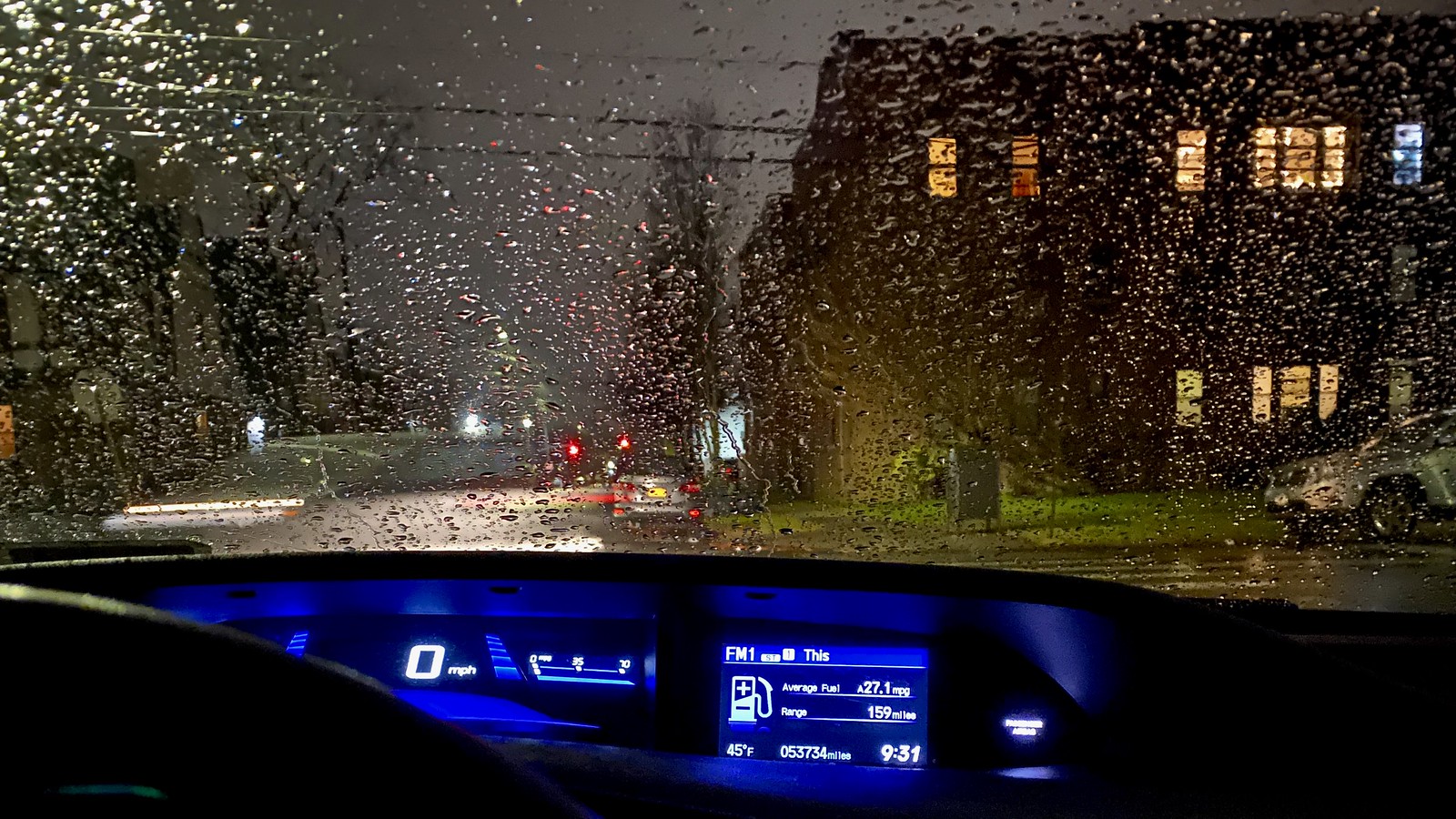The photograph captures the view from within a parked vehicle on a rainy night. The picture appears to be taken from a vantage point almost between the passenger and driver's seat, providing a clear view of the digital dashboard and the rain-soaked windshield. The dashboard, illuminated in a bluish hue, displays various details: 0 miles per hour, indicating that the car is stationary; an average fuel efficiency of 27.1 miles per gallon; a range of 159 miles; the odometer reading at 53,734 miles; a temperature of 45 degrees Fahrenheit; and a timestamp of 9:31 PM. Through the windshield, raindrops distort the view of the outside, where we see a dimly lit street with some parked cars, their red lights glowing in the rain. On the right side, a lit building with many windows can be seen, along with a grassy area and some trees in the background. The scene is framed with additional elements such as traffic lights, power lines, and a mailbox near the brightly lit building, emphasizing the stillness and the rainy, dark atmosphere of the night.